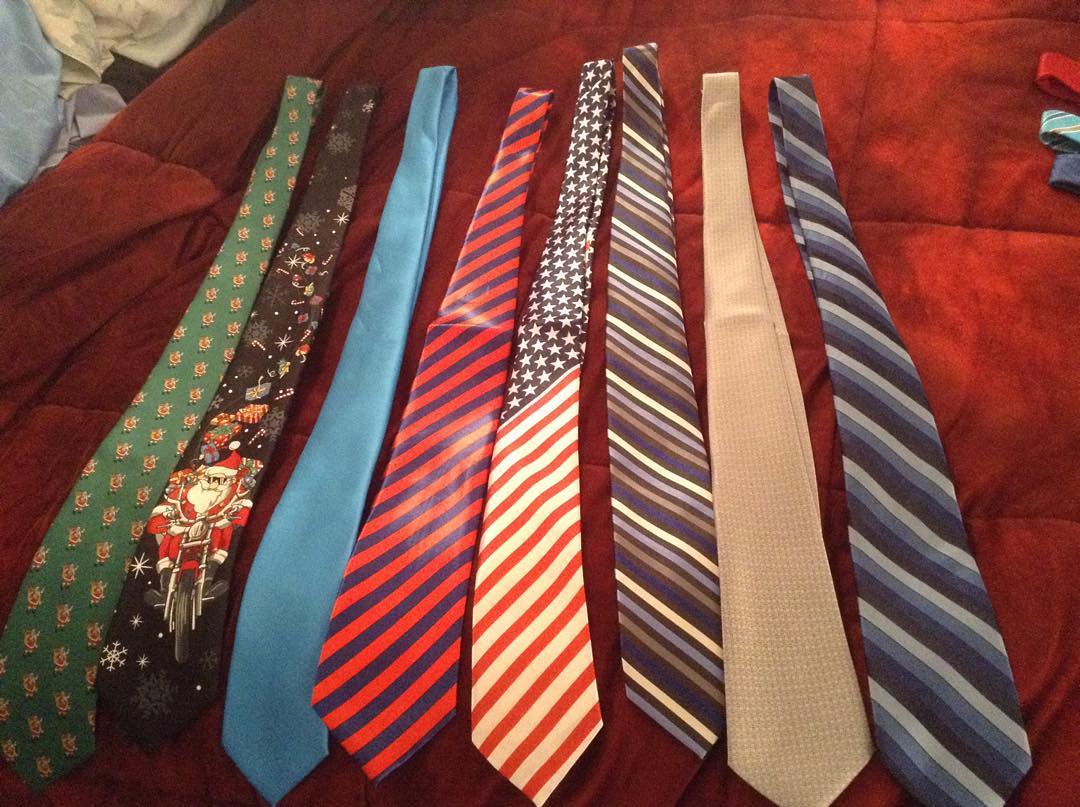This image is a photograph of a collection of eight neckties, arranged vertically on what appears to be a red comforter. The ties are displayed from left to right and exhibit a variety of colors and patterns. In the upper left corner, a blue and white cloth are visible, while the upper right corner shows the tips of three additional ties—red, dark blue, and light blue.

Starting from the left, the first tie is predominantly green with a repeating red and gold pattern. The second tie features a Christmas theme with a black background, showcasing a cartoon Santa Claus riding a motorcycle, surrounded by white snowflakes, stars, and candy canes. The third tie is a solid light blue. The fourth tie has shiny, even-width diagonal stripes in dark blue and red. 

The fifth tie resembles an American flag, with red and white stripes on the lower half and blue with white stars on the upper section. The sixth tie features diagonal stripes in brown, tan, and cream. The seventh tie is a tan color with a subtle waffle weave texture. The last tie on the right displays varying shades of blue and gray in diagonal stripes.

Overall, these ties appear somewhat dated due to their wide style, which is not currently in fashion.